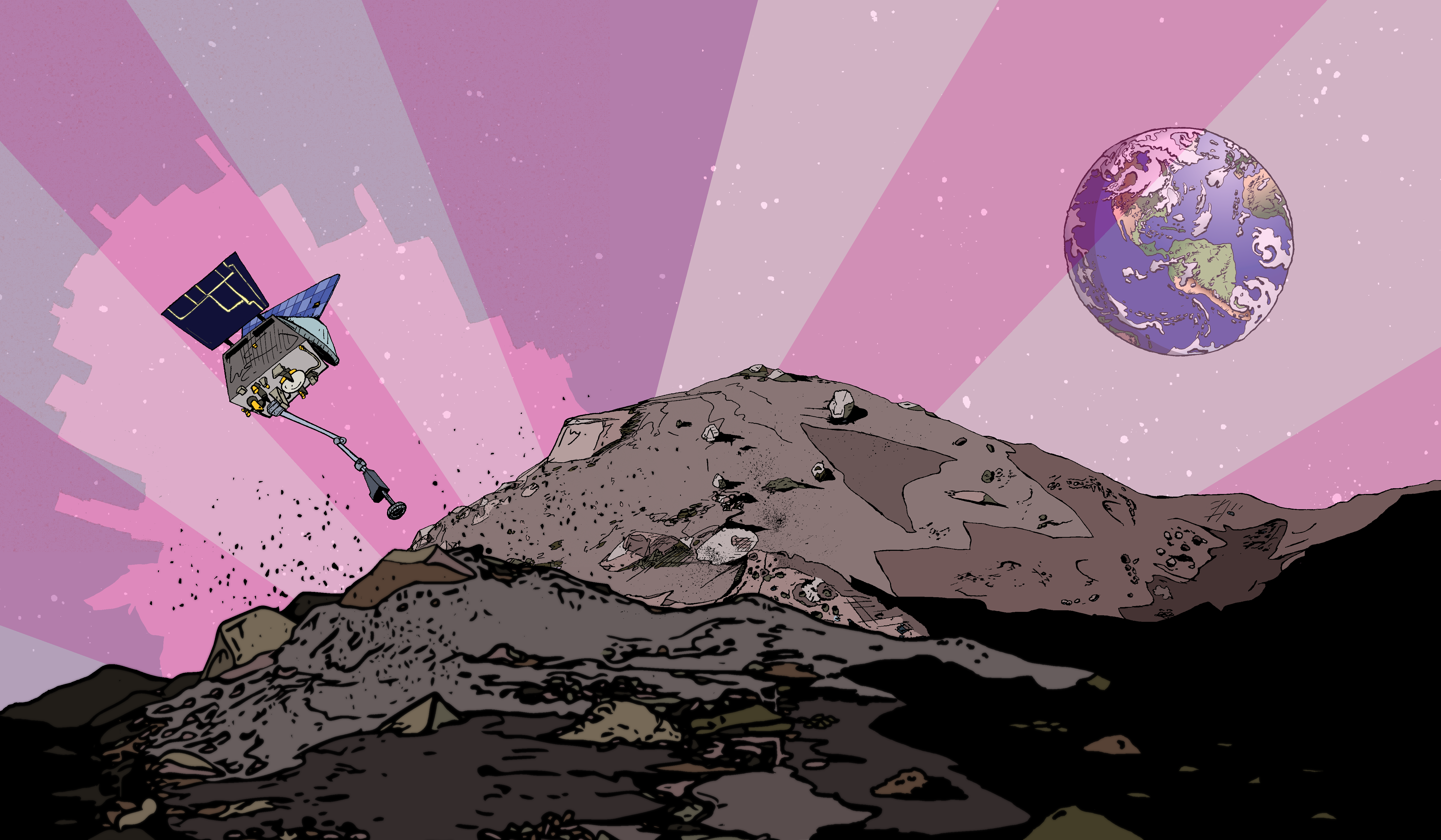A cartoon-style illustration presents a unique perspective, possibly set on the moon or a similar celestial body. The foreground is dominated by a mound of dirt and detritus in varying shades of brown, grey, and black, giving it a textured, earthy feel. Scattered within the debris are indiscernible, potentially man-made objects, adding an element of intrigue and perhaps a commentary on space waste or environmental issues. The background features alternating dark and lighter pink stripes in an arc pattern, evoking a surreal, otherworldly atmosphere. To the right, in the distance, is planet Earth, easily identifiable with its blue oceans, green continents, and swirling white clouds. On the left side of the image, a piece of technology that resembles a satellite floats above the mound. This satellite, depicted in dark grey with lighter-colored ports and switches, is equipped with solar panels that fan outwards; the panels are black with a yellow outline on the back and display shades of blue on the facing side. The overall composition blends a sense of desolation with subtle elements of color and technology, creating a thought-provoking visual narrative.